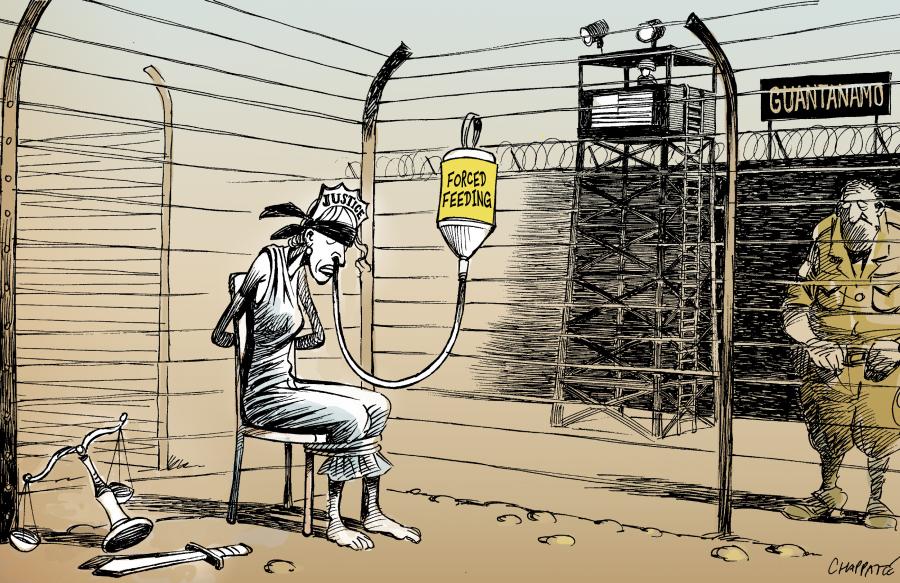The image is a detailed political cartoon set outside in the daytime, showcasing a prison courtyard with brown dirt and prison walls topped with barbed wire. Dominating the left-hand side of the image, there is a female figure resembling the Statue of Liberty, distinguished by her crown inscribed with the word "Justice." She is forcibly restrained to a chair; her hands are tied behind her back, and her legs are bound to the chair. A yellow tube labeled "forced feeding" is inserted into her nose, connected to a canteen.

To the right stands a soldier dressed in a khaki uniform, positioned under a black sign that reads "Guantanamo." In the background, a guard tower is visible. The scene captures a harsh, oppressive atmosphere enhanced by the political implications. At the bottom right corner, the artist has signed the piece with the name "Chappotte" or "Chappelle." The overall depiction highlights the theme of justice under duress, with the iconic symbol of liberty subjected to distressing treatment.